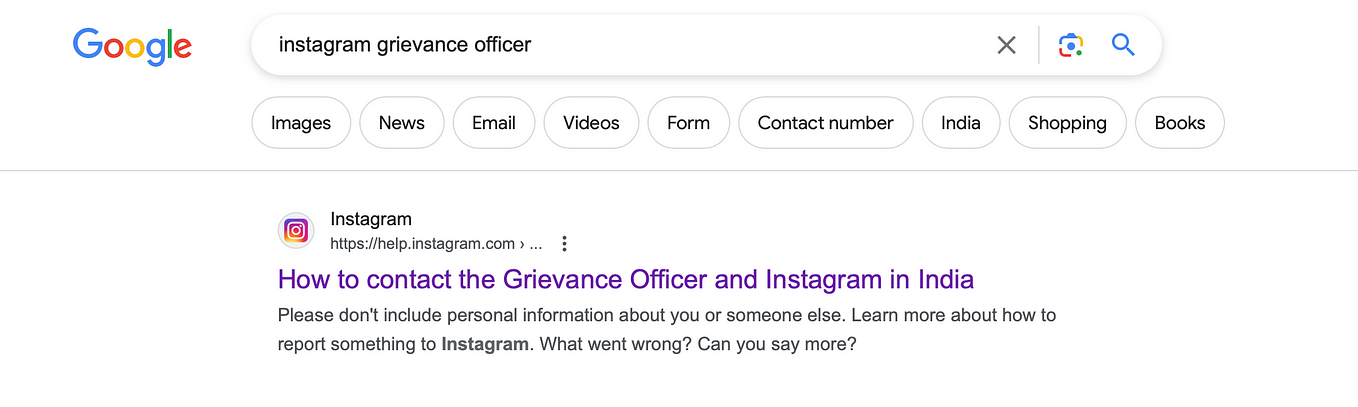This image displays a Google search results page. At the top left corner, the colorful Google logo features prominently, composed of two blue "G"s, two red "O"s, a yellow "O", a green "L", and a blue "E". Below the logo, the search box contains the query "Instagram grievance officer." Accompanying the search box are an 'X' icon, an image icon, and a magnifying glass icon.

Underneath the search box lies a horizontal menu with clickable tabs labeled: Images, News, Email, Video, Form, Contact Number, India, Shopping, and Books. Each of these tabs can be selected to refine the search results.

Following this menu, the results page features the Instagram name and icon, along with a partial URL ending in an ellipsis, indicating truncated web addresses. The main search result title, highlighted in purple, reads: "How to contact the grievance officer on Instagram in India."

Below the title, black text provides further details: "Please don't include personal information about you or someone else. Learn more about how to report something to Instagram." The word "Instagram" is bolded in this context. 

Additionally, there are prompts asking, "What went wrong?" and "Can you say more?" aimed at guiding users towards providing more specific information.